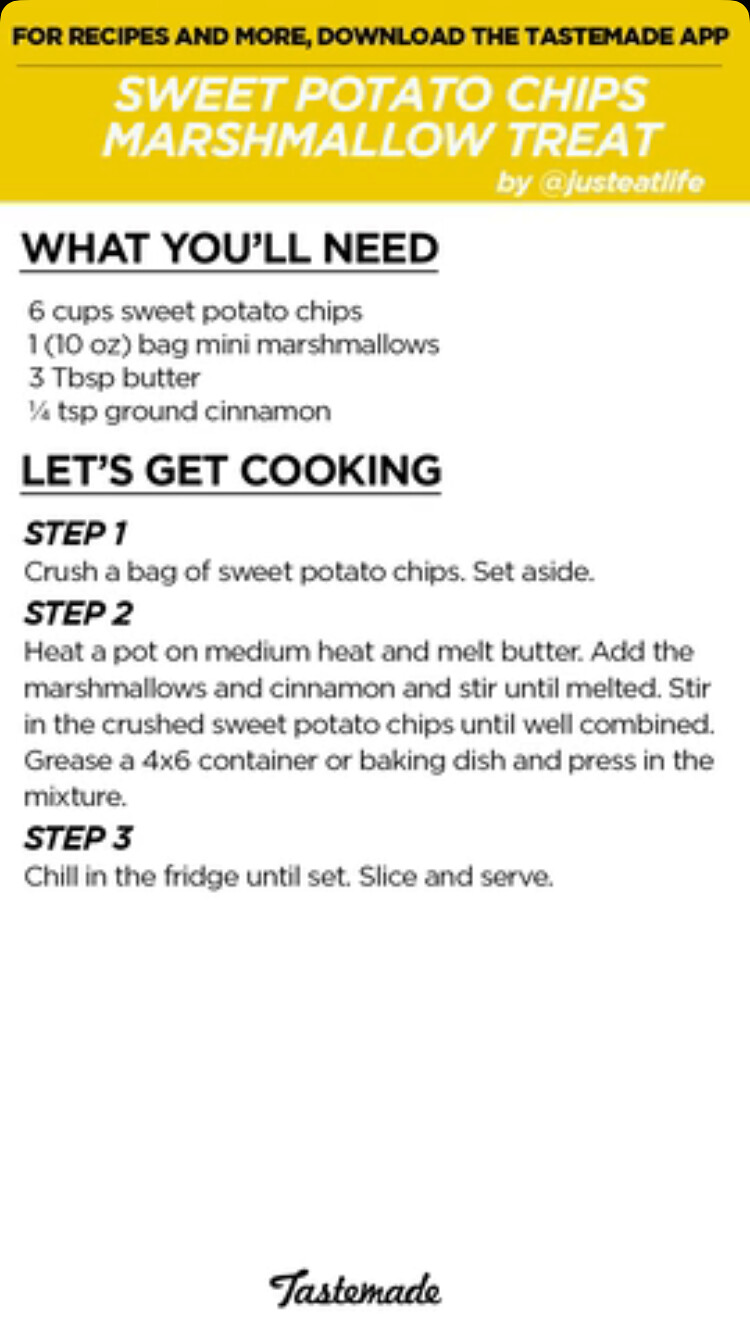The image features a detailed recipe for Sweet Potato Chips Marshmallow Treat. At the top, a yellow section displays the text in black, "For recipes and more, download the Tastemade app." Below it, in white letters on the yellow background, it says, "Sweet Potato Chips Marshmallow Treat," followed by "Buy at Just Eat Life." The subsequent section, in black text on a white background, is titled "What You Will Need" and lists the ingredients: six cups of sweet potato chips, one 10-ounce bag of mini marshmallows, three tablespoons of butter, and a quarter teaspoon of ground cinnamon. 

The "Let's Get Cooking" section proceeds with Step 1: "Crush a bag of sweet potato chips and set aside." Step 2 reads: "Heat a pot on medium heat and melt butter. Add the marshmallows and cinnamon, stirring until melted. Stir in the crushed sweet potato chips until well combined. Grease a 4x6 container or baking dish and press in the mixture." Step 3 instructs: "Chill in the fridge until set, slice, and serve." The bottom of the image features the word "Tastemade."

This comprehensive recipe guide is well-organized and emphasizes the sequence of steps needed to create the sweet, savory treat.